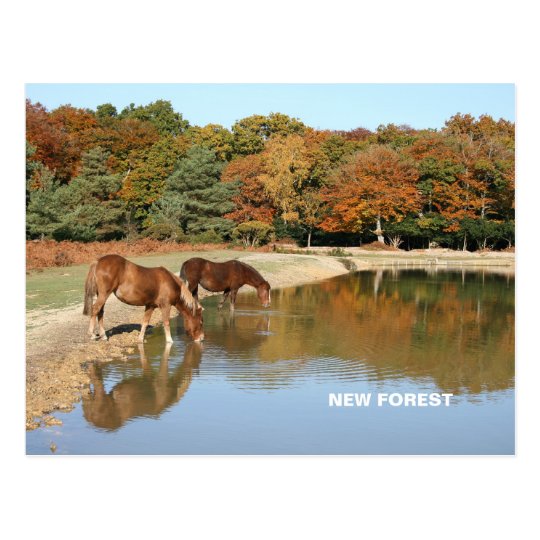In this outdoor midday scene set in the fall, two brown horses drink from a small body of water positioned centrally in the image. The horse in the foreground is a lighter brown, while the one in the background is a darker brown. The water shows ripples and reflections of their surroundings, which include tall, colorful trees transitioning into fall hues of green, yellow, and brown. The sky above is a bright, light blue, occupying a narrow band at the top. On the left, patches of grass interspersed with dirt stretch towards the trees. The text "New Forest" is visible in the center of the water. The overall setting appears to be a forested area, likely on a farm. The vibrant colors in the image include shades of blue, green, brown, tan, yellow, red, and gray, highlighting the natural beauty and serene atmosphere of the scene.